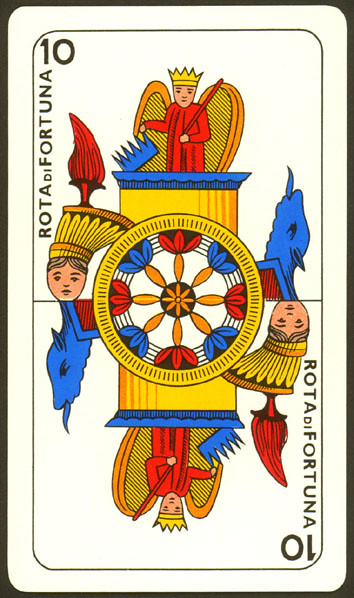The image depicts a Victorian-style playing card of standard size, featuring a white background. Central to the card's design are intricately imprinted or painted figures. At the top, a regal king is depicted standing on his throne, adorned with a gold crown and a red robe. He wields a red staff in his hand, symbolizing his authority. Beside him stands his queen, crowned with a grand golden headpiece that includes a tall red feather. 

A whimsical touch is added by a small blue goat positioned on the right side of the card, looking upward with its tongue playfully sticking out. The bottom half of the card mirrors the top half precisely, maintaining symmetry in the design.

In the top left corner, the number "10" is displayed, accompanied by the text "Roda de Fortuna," suggesting elements of fortune or destiny, possibly in a foreign language. The card overall presents a detailed and elegant Victorian aesthetic.